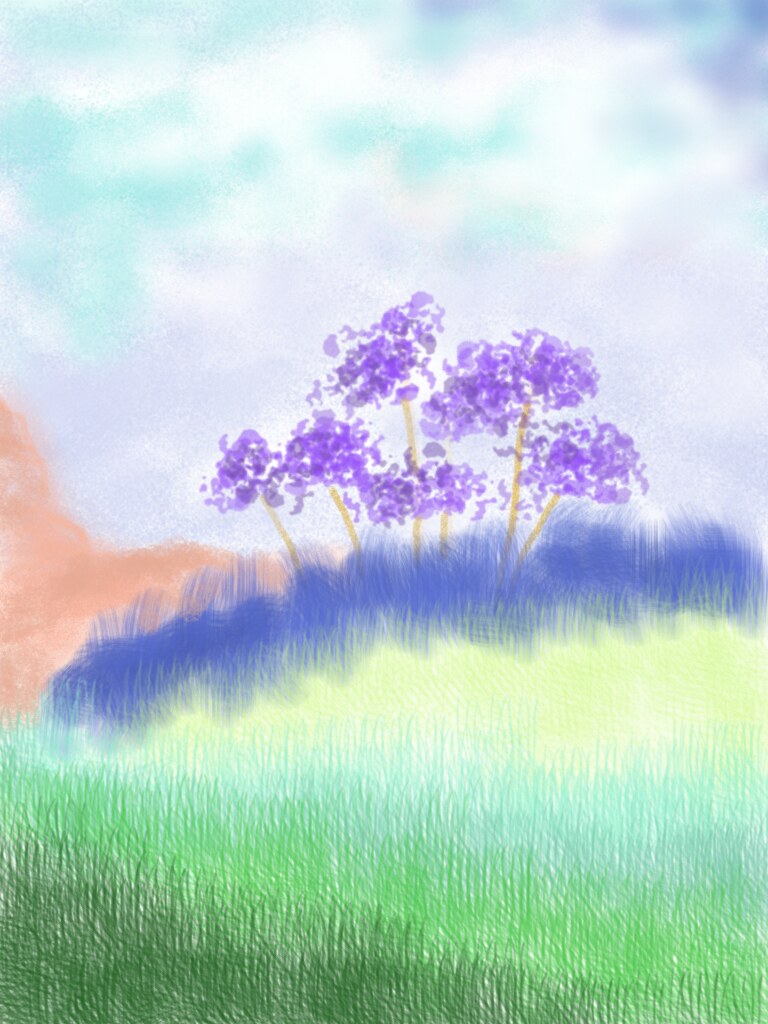This artwork, seemingly created using colored pencils and watercolors, presents a rich and vibrant landscape. At the base of the image, dark green grass blankets the ground, gradually transitioning into lighter green hues as the terrain ascends a gentle hill. Midway up the slope, the grass takes on a bluish-green tint, eventually evolving into a mint green shade near the top. A striking horizontal blue strip traverses the peak, resembling a patch of grass. Embedded in this gradient are numerous yellow stems, each topped with delicate purple flowers, adding a dash of lively contrast. 

To the left of the hill, a prominent red rock formation introduces a rugged texture to the scene. Above it all, the sky progresses from a light blue expanse mingled with splashes of white, to very light lavender clouds, creating a serene and airy atmosphere. The combination of colors and natural elements gives the artwork a sense of depth and tranquility, beautifully capturing the essence of an imaginative landscape.